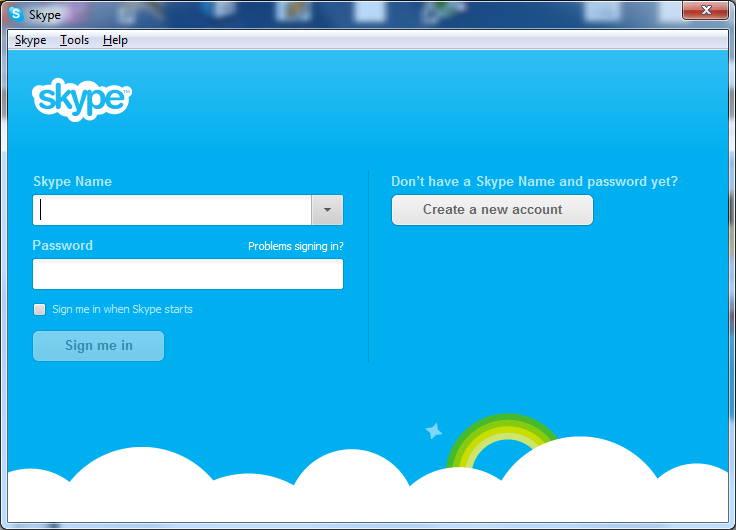The image is a screenshot captured from a computer, displaying the Skype login interface. The upper portion of the image is slightly blurred, with the Skype logo and name in black clearly visible in the upper left-hand corner. 

Icons in the background appear blurry, but are recognizable. In the upper right-hand corner, the characteristic red 'X' button for closing the window is visible. Just below this, there is a gray rectangular menu bar with black text options labeled 'Tools' and 'Help'. 

The main interface has a sky blue background. Prominently on the left side, 'Skype' is displayed in larger text. Below it, prompts for 'Skype name' next to a white search bar are visible, accompanied by a gray button for additional options. 

The password input field and a link labeled 'Problem signing in?' are situated below it. A checkbox labeled 'Sign me in when Skype starts' is present, and the 'Sign me in' button is shown grayed out, indicating the necessary information has not been filled out yet.

A vertical line separates the left side from the right side, which features a prompt: 'Don't have a Skype name and password yet?' A gray button invites users to 'Create a new account.'

At the bottom of the screen, there is an artistic illustration with fluffy white clouds, a small star, and a partial rainbow colored in shades of yellow and green.